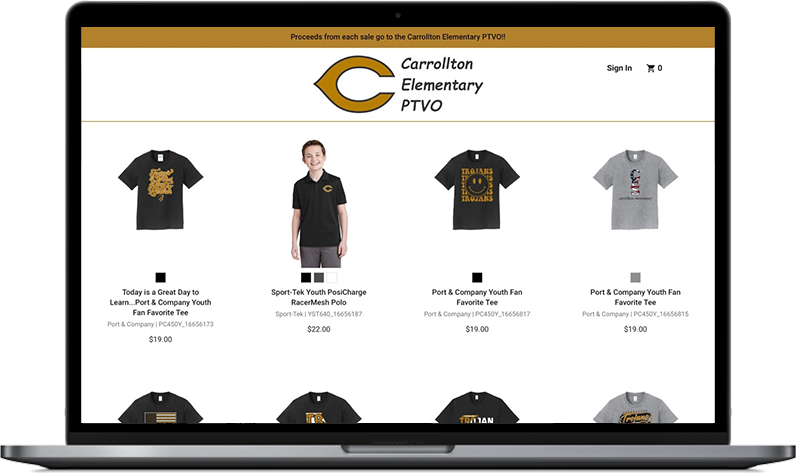The image showcases a mock-up of a storefront website displayed on an open MacBook with a sleek metallic silver body. The website is dedicated to Carrollton Elementary PTVO, featuring their logo—a gold "C" outlined in black, with the left side tapering to a point, giving it a leaf-like appearance. 

At the top of the webpage, a gold bar prominently displays the message "Proceeds from each sale go to the Carrollton Elementary PTVO" in black font. The site appears to be offering school merchandise, specifically various types of clothing.

Visible products include:
1. A black t-shirt with gold lettering that reads "Today is a great day to learn" – identified as a Port & Company Youth Fan Favorite Tee, priced at $19.
2. An image of a boy modeling a polo shirt featuring the leaf-like "C" logo – described as a Sport-Tek Youth PosiCharge RacerMesh Polo, priced at $22.
3. Another black t-shirt with gold lettering and a black smiley face – also listed as a Port & Company Youth Fan Favorite Tee, priced at $19.
4. A heather gray t-shirt with the "C" logo emblazoned with an American flag design – yet another Port & Company Youth Fan Favorite Tee, priced at $19.

Below these items, additional black and gray shirts are visible but partially cut off, making the details difficult to read. The overall design of the website is cohesive and clearly aimed at promoting school spirit through branded apparel.